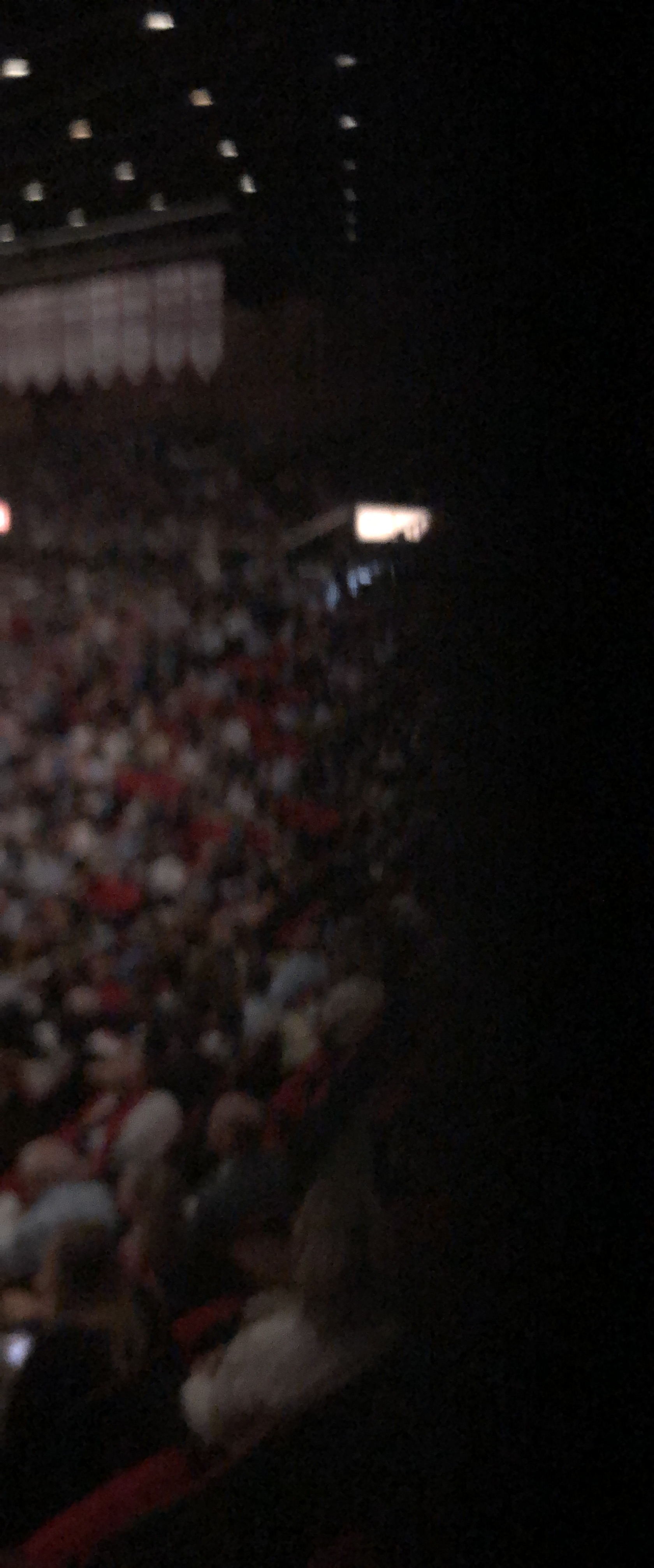This is a blurry, vertically-oriented image likely taken from inside an indoor arena during an event. The scene captures a crowded audience sitting in rows of red seats, all facing towards the left-hand side of the picture. The general atmosphere suggests it could be a concert or a show, though there is an impression of a repurposed sports arena due to the observed banners and stadium lighting. The banners, white with red borders and lettering, hang from the top, reaching downwards. Circular lights are mounted across the ceiling, casting illumination predominantly on the left side of the image. There is also an exit area lit up, possibly guiding attendees to their seats. The right half of the image is entirely black, as though obscured by an object or shadow. The crowd seems to comprise people in varied colored shirts, and their blurry forms suggest a mix of older individuals. The overall scene exudes a sit-down, observation-focused gathering.